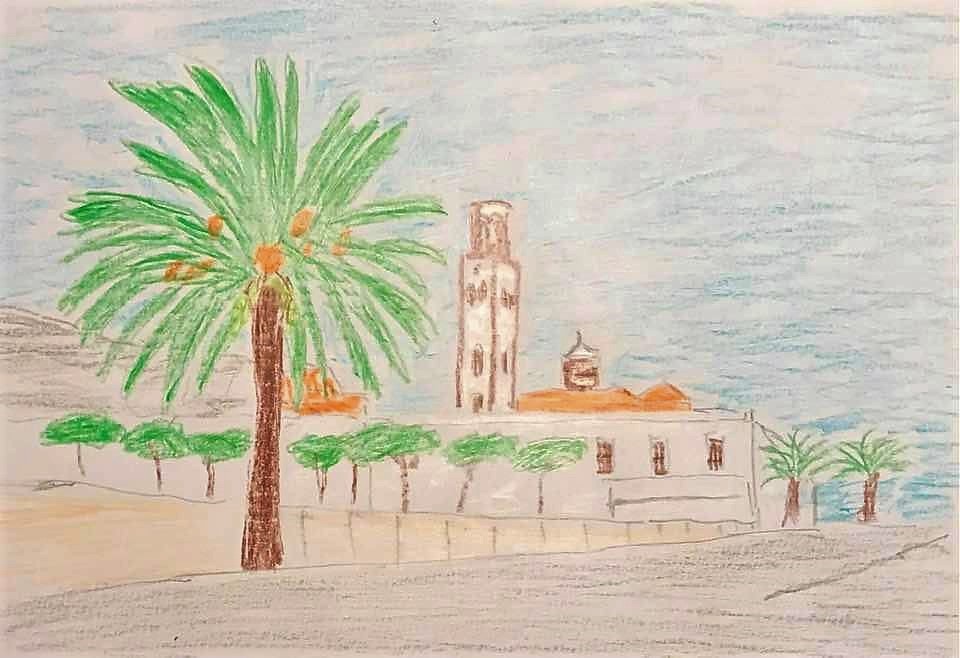The image showcases vibrant colored pencil drawings, with a detailed and dynamic composition. Intricate blue scratch marks adorn the top right corner, spreading across the background to add texture. A prominent clock tower stands tall in the center, embellished with shades of white and brown. To the right of the clock tower, a large rooftop in bright orange catches the eye. In the background, lush green leaves and sturdy brown trunks hint at a dense foliage. Two stately palm trees rise to the right of the scene, their fronds reaching skyward. The foreground features stark black shading, defining the ground, while a sunny yellow sandy beach stretches across the left side. Dominating the front is a majestic palm tree, complete with a large branch, clusters of coconuts, and a burst of green leaves. The background continues the theme of verdant green leaves interspersed with brown trunks, creating a cohesive and lively natural setting.